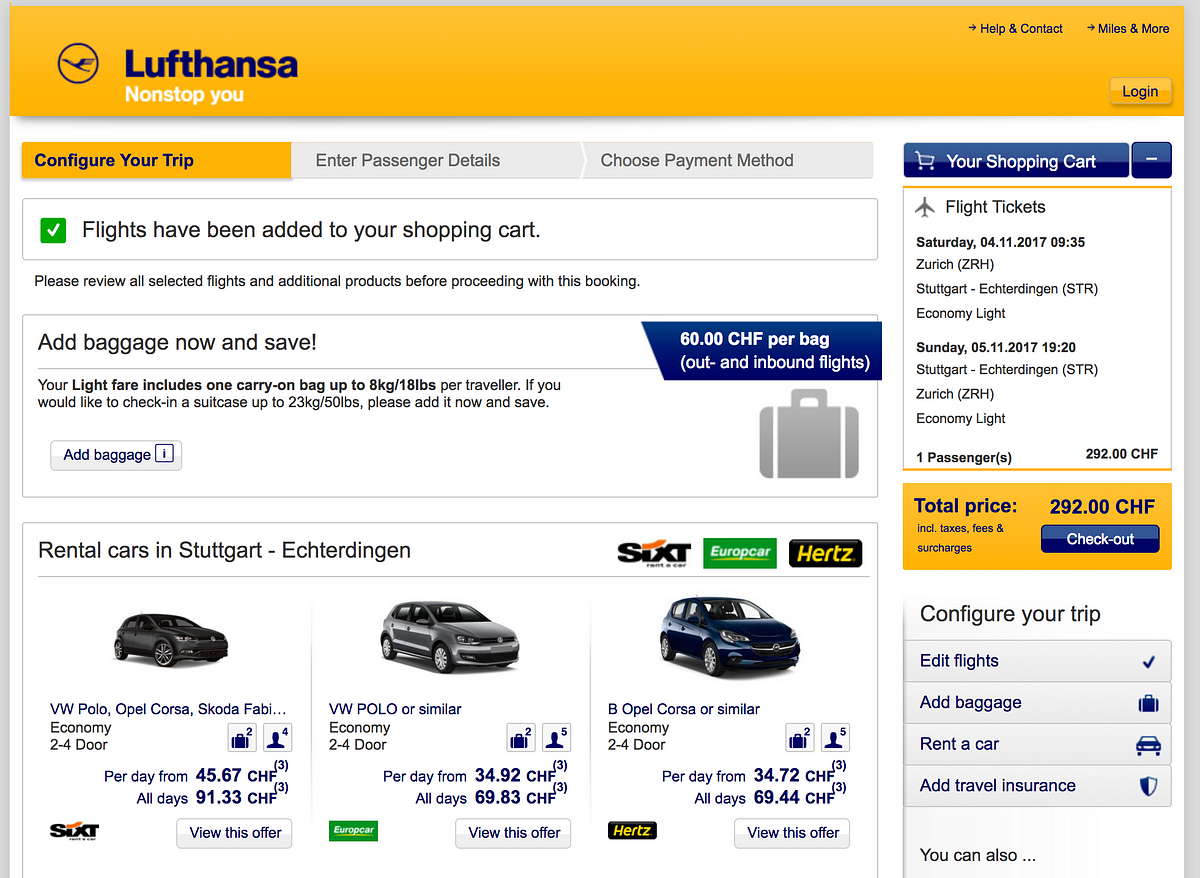This vertically oriented image appears to be a screenshot from a travel booking website, potentially accessible via a computer. The webpage has a visually distinct gray border that encompasses the entire image except for the bottom edge, where it merges with the white background of the screen.

At the top of the webpage, a vibrant orange banner displays the logo on the upper left side, accompanied by the text "Lufthansa, nonstop you." The upper-right section features links for "Help and Contact," "Miles and More," and a "Login" button positioned just below these options.

Transitioning from the orange banner, the central portion of the page shifts to a clean white background. On the left side, the navigation menu highlights "Configure Your Trip" in orange, indicating the current step in the booking process. Other options such as "Enter Passenger Details" and "Choose Payment Method" are visible but not selected.

Below this, a notification assures the customer that "Bags have been added to your shopping cart" and urges a review of all selected flights and additional products before proceeding with the booking. A promotional message states that adding baggage now can save the customer 60 CHF per bag for both outbound and inbound flights. The fare includes one carry-on bag weighing up to 8 kilograms (18 pounds) per traveler. For those needing more luggage, there is an option to add a checked suitcase up to 23 kilograms (50 pounds) and save on fees.

Further down, there is an illustrated clipart of luggage and information about rental cars available in Stuttgart. Options from rental companies such as Sixt, Europcar, and Hertz are presented, allowing users to view their offers and select based on preference.

On the left side of the screen, a shopping cart summary displays the total price, providing a straightforward way to review and proceed to checkout.

Overall, the page effectively guides users through configuring their trip, adding necessary extras, and finalizing their booking.